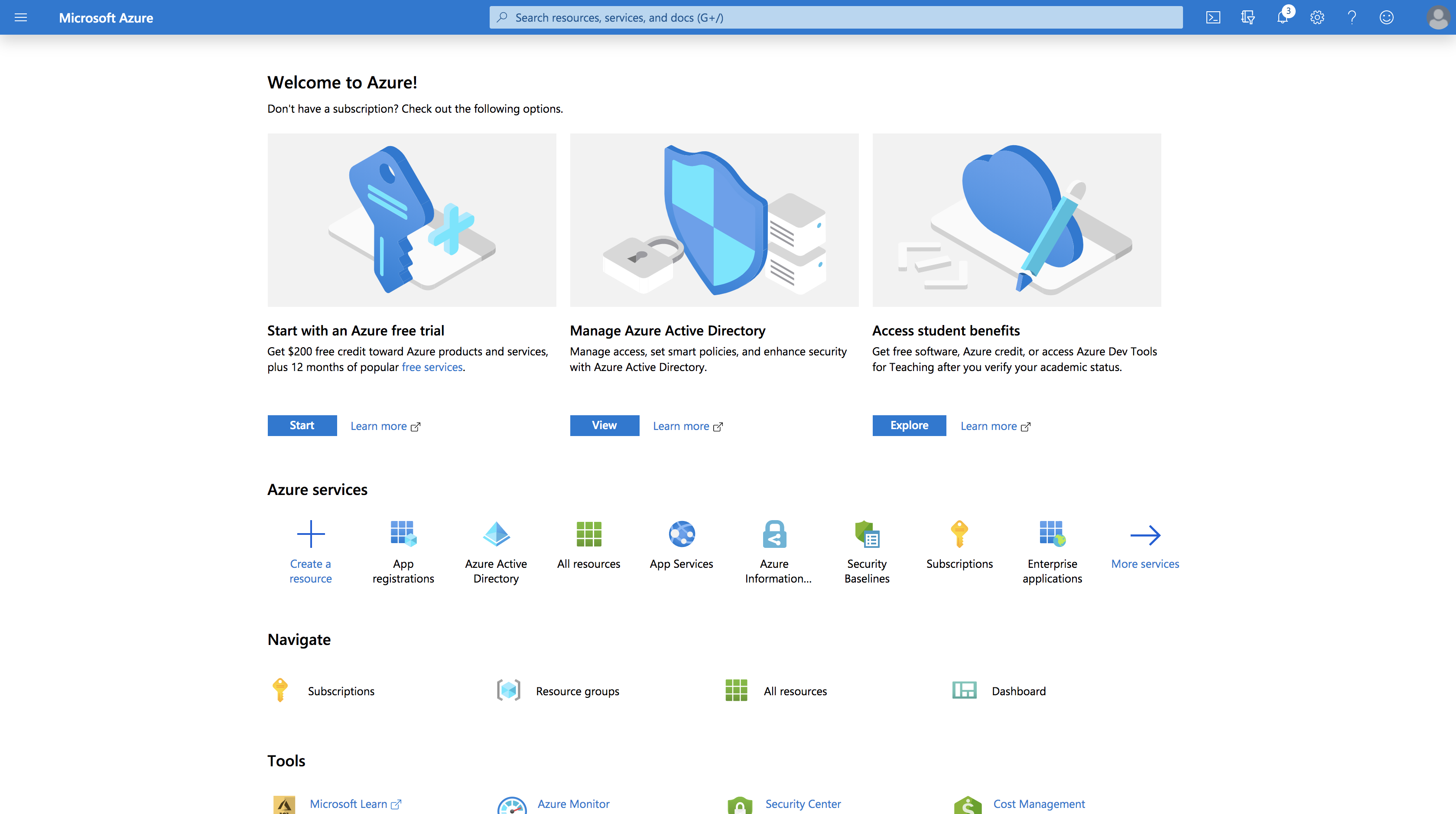This screenshot of a website features a top dark blue header approximately half an inch in height, transitioning to a white background below. In the top left corner of the header, three small gray lines serve as a menu icon. Directly to the right, the word "Microsoft" appears in white.

In the center of the header, there is a light blue search bar. Adjacent to the search bar on the right, a small square contains a greater-than sign pointing left. Following this are several icons: a square emblem, a notifications icon featuring a white circle with the number "3" inside, a settings icon, a help icon (question mark), a friends icon, and finally, a profile icon in the far right corner.

Just below the header, about two inches from the left margin, the text "Welcome to Azure!" is written in black. Beneath this, smaller black text reads, "Don't have a description? Check out the following options." Under this text are three squares, each containing distinct images and descriptions:

1. The first square on the left has a blue key icon with the text "Start an Azure free trial" beneath it.
2. The center square features a blue shield icon labeled "Manage Azure Active Directory."
3. The rightmost square shows a blue cloud icon with the label "Access student benefits." Below each title are two lines of information and a blue tab that says "Learn more."

Further down, the section titled "Azure Services" in black text is followed by nine icons arranged left to right, concluding with a blue arrow pointing right accompanied by the text "More services."

Below this, the heading "Navigate" in black is followed by a row of four icons. The section under this is labeled "Tools," also in black, and contains another row of four icons.